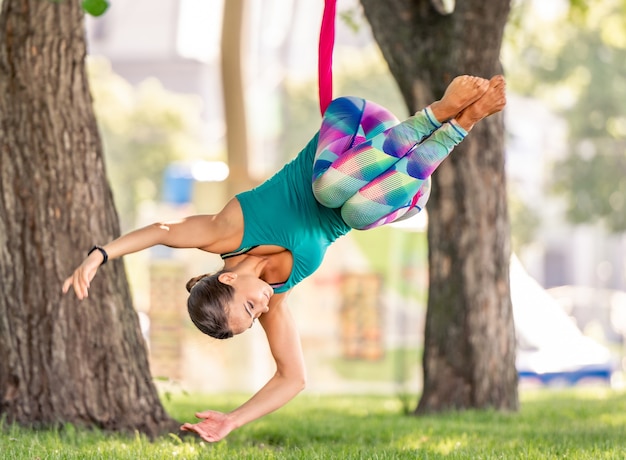In this photograph taken outdoors, likely in a city park, a woman is captured in the midst of practicing fly yoga or bungee yoga. The scene is set with green grass and a couple of trees in the background, along with an out-of-focus cityscape in the distance. The centerpiece of the image is the woman, who appears to be hanging upside down at a diagonal angle, supported by a bright red strap connected to a tree above her.

She is attired in a tight-fitting, aqua-colored tank top and vibrant, full-length leggings adorned with geometric shapes in a spectrum of colors including blue, purple, green, white, yellow, and red. Her dark hair is neatly pulled back into a bun, and she sports a watch on her left wrist. Barefoot, her right hand grazes the top of the green grass, while her arms extend gracefully above her head. Her head is pointed towards the ground, tilted slightly to the left, and her toes are directed towards the top right corner of the image, creating a striking, dynamic pose.